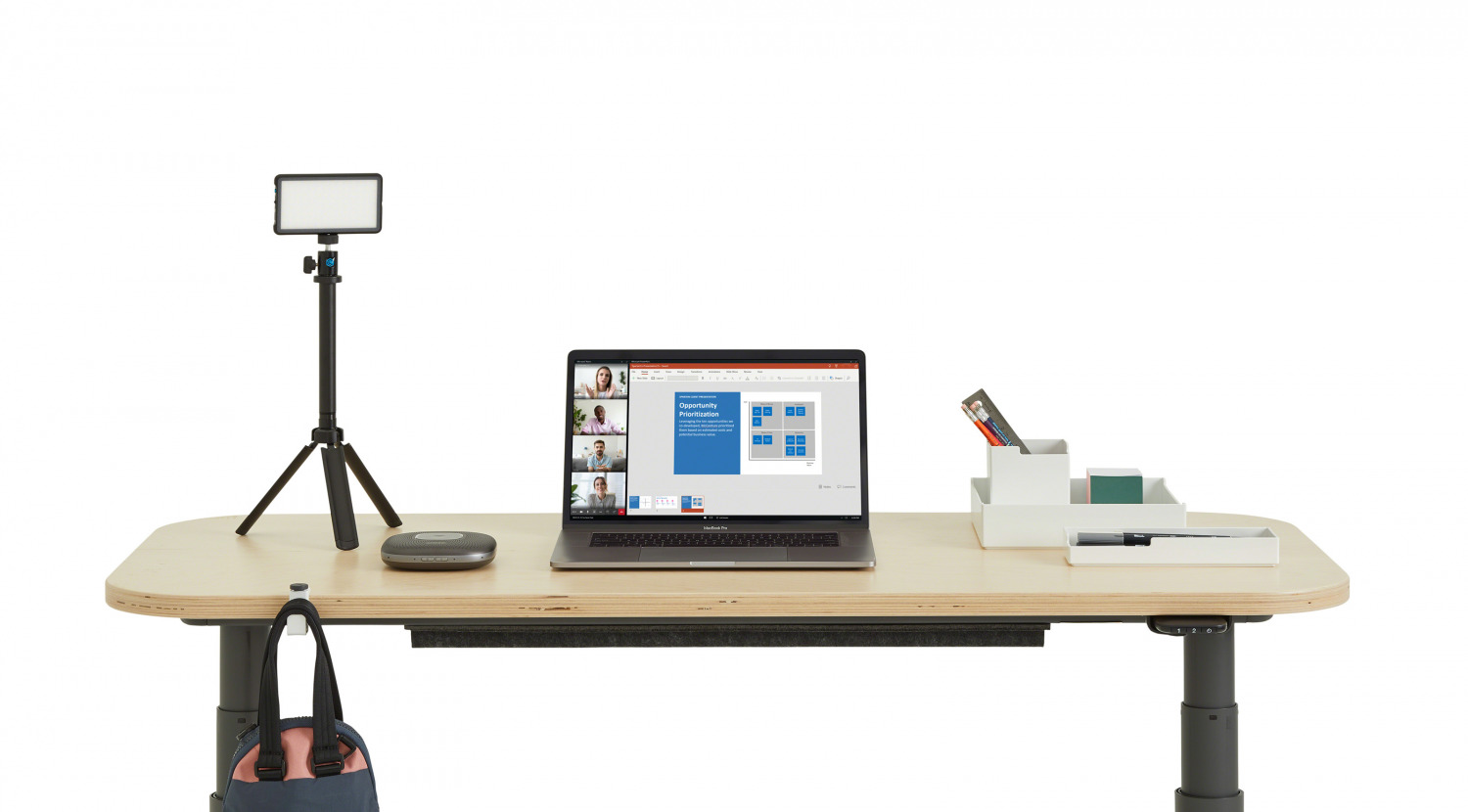The image depicts a minimalist desk setup with a clean, white background. The desk itself is equipped with large, dark gray steel legs, potentially adjustable as suggested by the buttons on the right leg, allowing the desk to rise and lower. The tabletop is a light pine wood with rounded edges, contributing to a sleek appearance. At the center of the desk is an open laptop displaying a Zoom meeting interface, showing several participants on the left of the screen along with some text and diagrams in blue and gray boxes.

On the left side of the desk, there's a tripod holding a smartphone in a horizontal position, with a round, black case placed nearby. To the right of the laptop is a white desk organizer containing a notepad, writing utensils, and a block of green sticky notes. A brown bag with black straps and a pink curved detail is hung from a white hook on the front of the desk, adding a functional yet stylish touch to the organized workspace. Overall, the setup exudes a professional and tidy aesthetic.